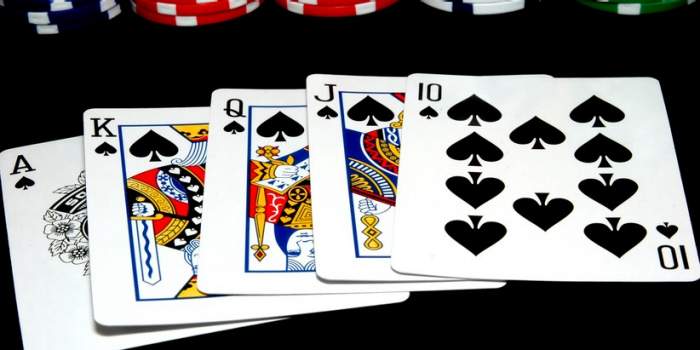Against a sleek black background, a series of poker chips and a remarkable poker hand are prominently displayed. The poker chips are lined up horizontally along the top. Starting from the left, the first chip is dark blue with small white rectangles. Next to it, there are two consecutive red and white chips, followed by a white chip with small black rectangles. The sequence ends with a green and white chip to the far right.

Below the chips is an impressive poker hand, laid out from left to right: the ace of spades, followed by the king, queen, jack, and ten of spades. This hand, known as a royal flush, is the highest possible hand in poker, making it exceptionally valuable. The intricate details on the chips highlight their main colors, with the small rectangles contrasting beautifully against the primary hues. The subtle variations in chip patterns and the pristine arrangement of the cards create a visually striking tableau that emphasizes both the elegance and excitement of the game.